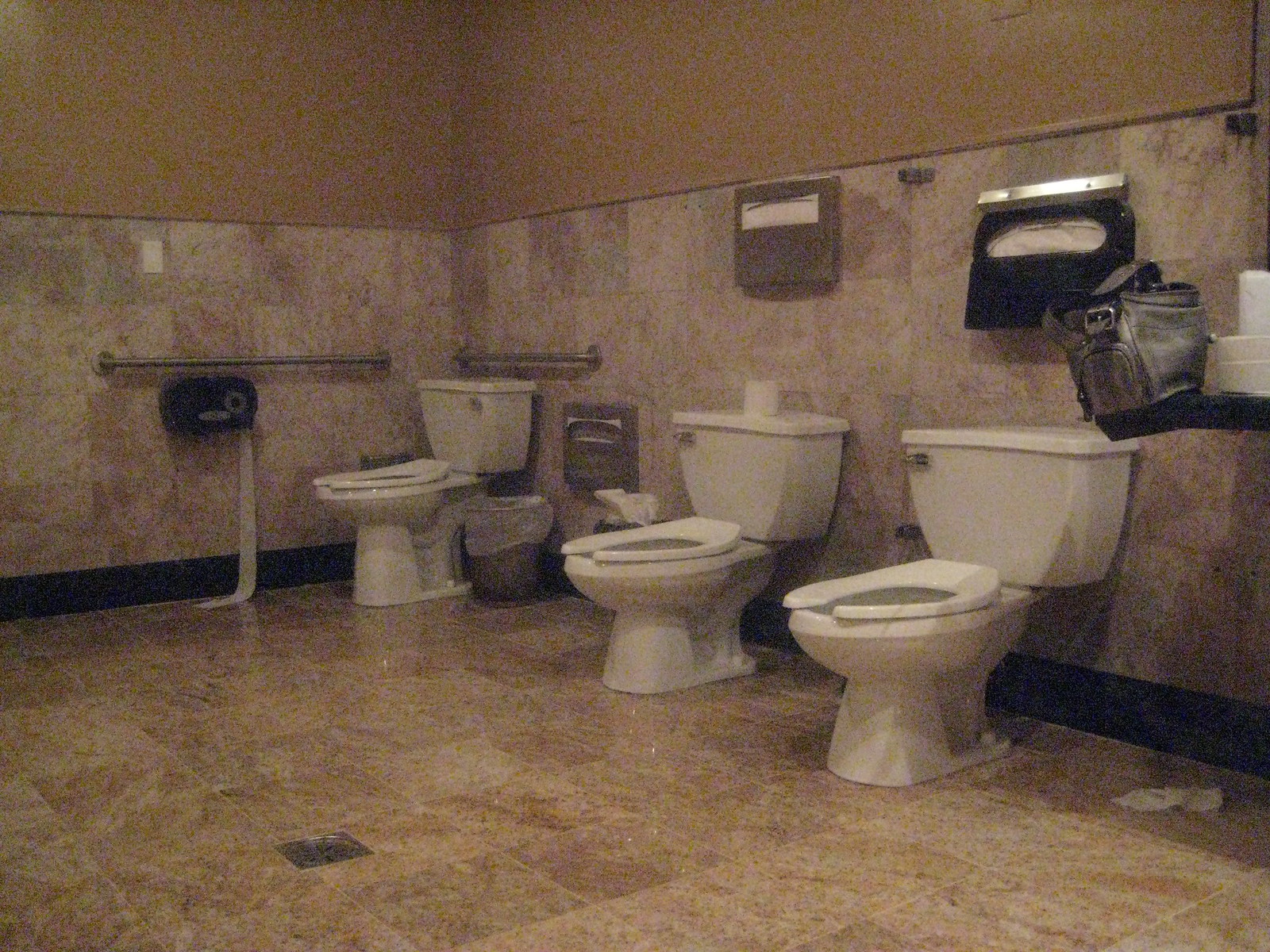This is a photograph taken inside a public bathroom, characterized by its brownish-tiled floor and matching half-wall tile, which transitions to a dark beige or yellowish upper wall. The grainy image captures three white porcelain toilets aligned from left to right. The leftmost toilet, likely designated for handicapped access, features safety rails and a trash can beneath it. A roll of toilet paper is placed on the back of the middle toilet, while the rightmost toilet has a metal tissue dispenser above it. To the right of the farthest toilet is a white shelf holding a black leather bag. Scattered items of trash and a long piece of toilet paper reaching the floor add to the scene's untidiness.